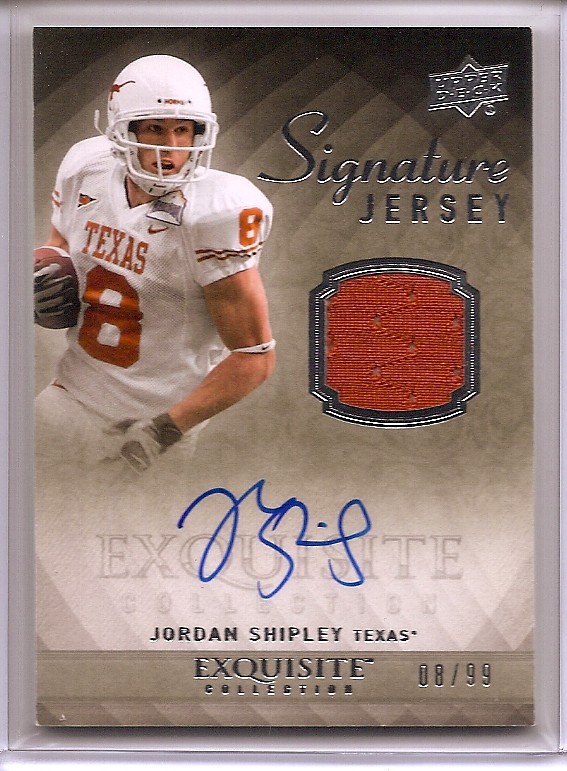The image showcases an Upper Deck Exquisite Collection football card encased in a plastic protective case. The card prominently features Jordan Shipley, a Texas football player, wearing a white Texas jersey with the number 8 visible on both his chest and shoulder. Shipley is depicted in action, holding a football in his gloved right hand, with his body angled diagonally and his helmeted head turned to the right. His facial expression is captured vividly with open eyes and mouth, all beneath the helmet’s face guard.

In the background of the card, the words "Exquisite Collection" are displayed. A red, sequined symbol with a silver border is also visible, contributing to the textured and patterned silver backdrop of the card. The text "Upper Deck Signature Jersey" appears on the right side of the card, highlighting its exclusivity. The card is hand-signed by Shipley in blue marker, with his signature partially overlaying the “Exquisite Collection” text. The card is marked as 08/99, indicating its limited edition status.